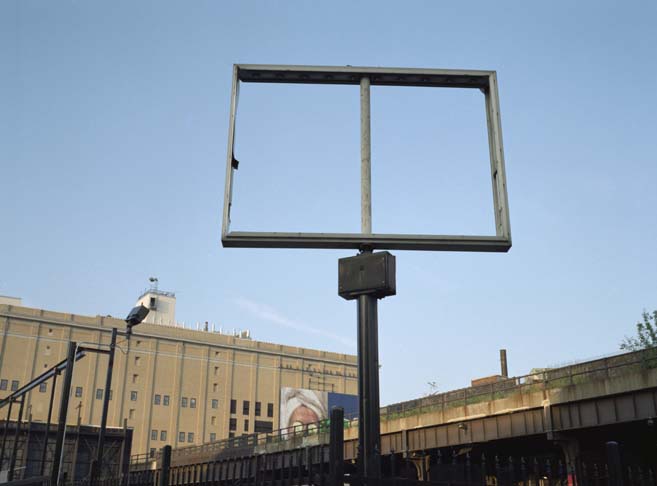The image depicts an old wooden sign set within a weathered wooden frame. The sign itself, which once included an insert, is now bare and composed entirely of wood. The structure is supported by a central wooden pole. Positioned above an overpass to the right, the scene includes a billboard featuring a woman with a head wrap and cucumber slices over her eyes, while the adjacent billboard has a navy background but is otherwise indistinguishable. Nearby are steel buildings, adding an industrial touch to the area. The underside of the overpass shows visible rust. In the background lies a large, tan factory-like building, its imposing silhouette highlighted by a single smokestack against a blue sky adorned with a scattering of clouds. The entire composition evokes a blend of decay and industrial progress, set against a serene sky.